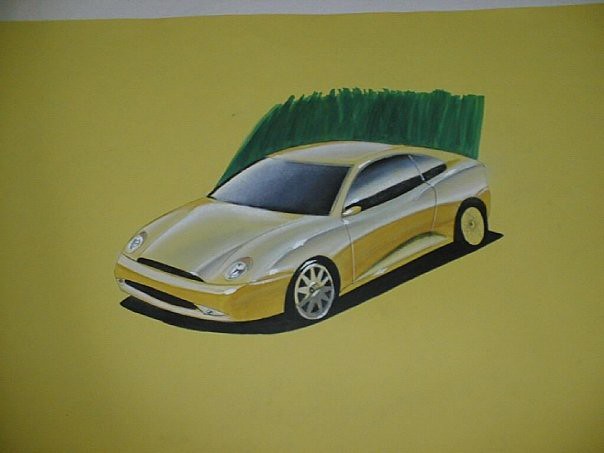This image appears to be a child's art project, featuring a sports car drawn with a mix of yellow and silver colors. The background is predominantly a mustard yellow sand or ground with a gray sky at the horizon. The car itself exhibits an unusual artistic style, with inconsistencies like a silver hubcap on the front wheel and a yellow hubcap on the back wheel. Both the windshield and side windows are colored black and show no interior details. Behind the car is a peculiar green bar, shaded to resemble tall grass or a hedge, although it appears more like a single blade of grass due to its narrow width. There are also white streaks on the car and a black shadow beneath it, adding to the ground effect.